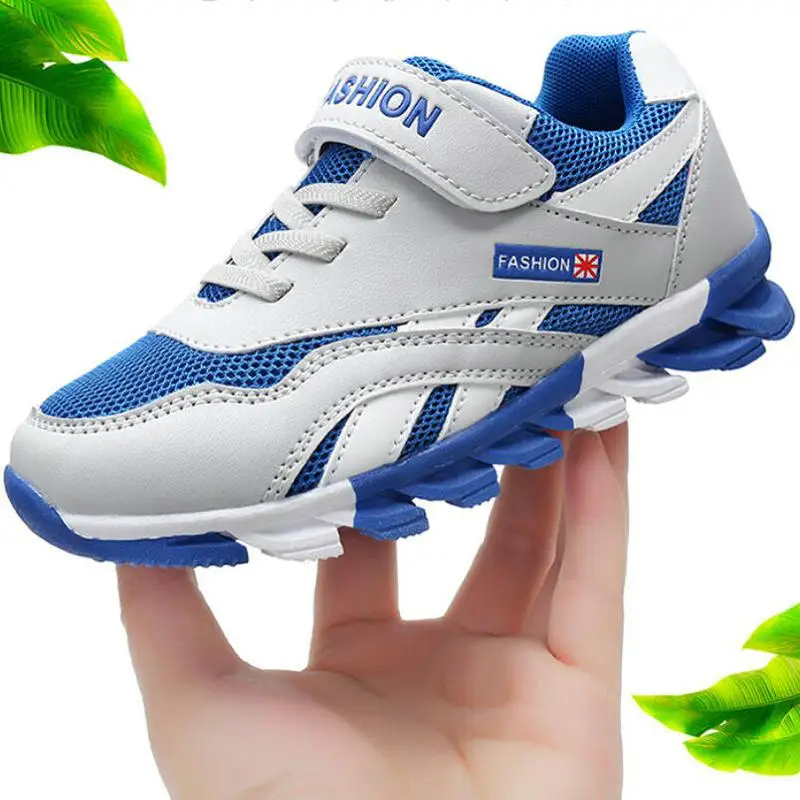In this detailed image, a woman's hand is holding up a blue and white athletic sneaker, which appears to be designed for running. The sneaker prominently features a blue mesh fabric on the front and sides, with alternating blue and white soles. The upper includes a distinctive Velcro strap that displays the word "Fashion" in blue letters, along with a red sign that resembles hieroglyphics, catching the eye. White shoelaces secure the shoe, and there is an additional blue tag on the side which also bears the word "Fashion" and features a small flag-like symbol, possibly Japanese. Details such as visible stitching on the white part and a high back against the heel further highlight the shoe's design. The scene is framed by green leaves, with two leaves positioned in the upper left corner and three in the lower right corner. The backdrop is a clean white, emphasizing the sneaker and the hand that holds it.